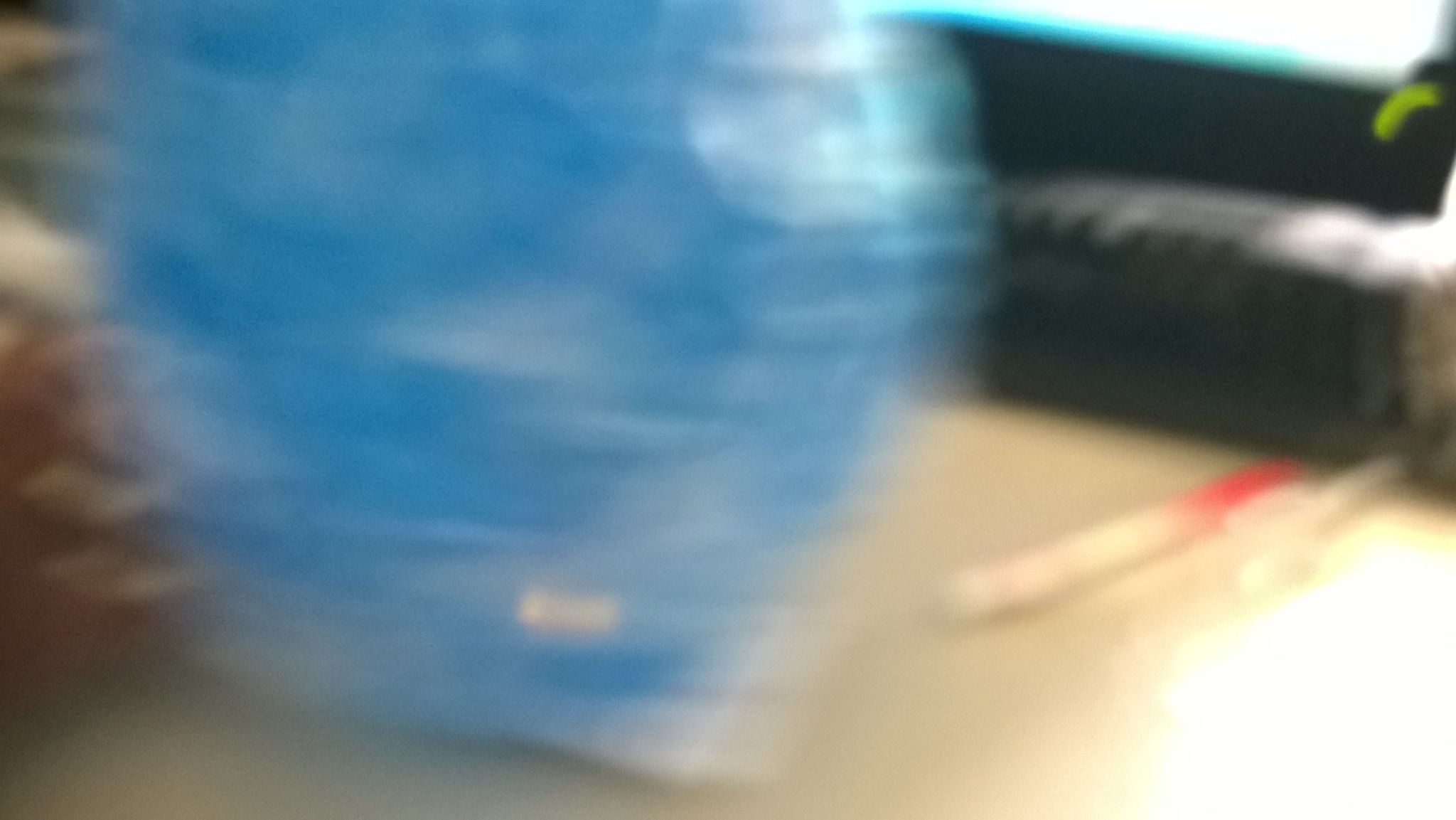In this extremely blurry photograph, a large, vivid blue sphere with wisps of white appears centrally. The surface of the sphere is glossy, showing reflections including a white bubble at the top right and a white rectangular shape at the base. The sphere sits on a light-colored surface, possibly a tan tabletop or floor, with light reflecting off it creating a glare in the bottom right corner. To the right in the background, there is a black, reflecting object that could be a leather couch or an oversized chair. Additionally, there seems to be a leaf of a plant nearby and some small objects, possibly a pen with a red cap and a tiny pair of scissors next to the sphere-like shape. Though the exact details are hard to discern due to the extreme blurriness, these elements provide a tentative composition of the scene.